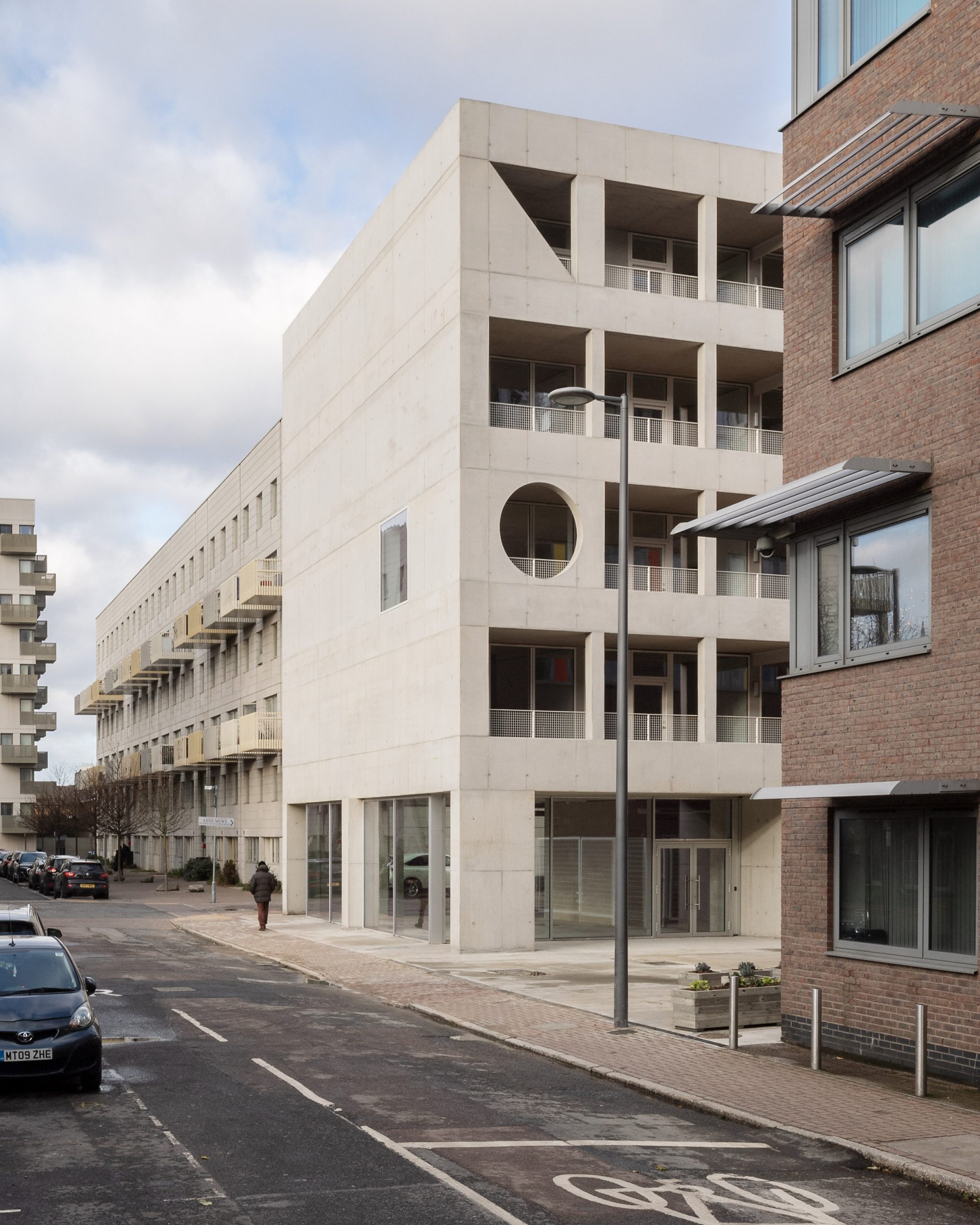This photograph captures a street scene taken from slightly above street level. In the bottom left of the image, a black road with white markings, including a bicycle symbol, can be seen. Several cars are parked along the sides of the road, with no vehicles in motion. On the right side of the road, a sidewalk features a person walking, and beyond this sidewalk are several large, multi-story buildings. The nearest building on the right is constructed from brown-colored bricks, and just beyond it, there is a cream-colored building featuring patios with white railings on each balcony. Further back, there's another large white building with balconies painted in various shades of gray, white, and beige. The bright blue sky above is dotted with white clouds, enhancing the overall clarity and brightness of the setting.